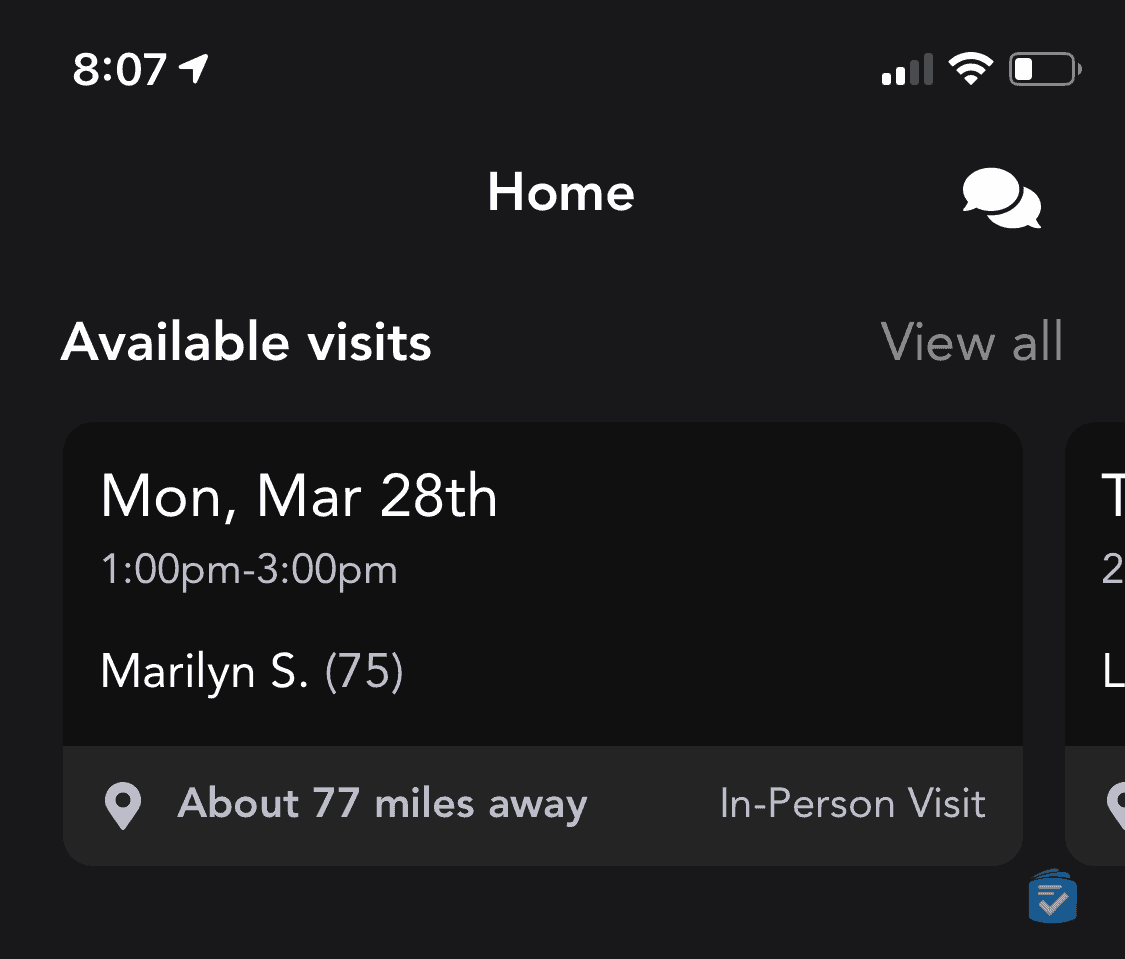A detailed screenshot captures a mobile interface, possibly enlarged for clarity. The top status bar shows a timestamp of 8:07, with two Wi-Fi bars and a battery at approximately 35%. Below this, the text "Home" is displayed, alongside two speech bubbles on the right, signaling a chat application. 

The central area features options titled “Available Visits” and “View All” on a dark gray background. Beneath these options are floating fields in darker gray with a lighter gray footer across the bottom. One prominent section provides details for an appointment on "Mon, Mar 28th". 

The details include:
- A blue text indicating the time slot: "1 p.m. to 3 p.m." (with p.m. in lowercase).
- A white text, "Maryland S.", followed by a light gray "75" enclosed in brackets.

The footer includes a map icon and the text “About 77 miles away” on the left, with the notation “In-person visit” on the right. Additionally, a white check mark on a blue field appears below these tiles.

Overall, the structured layout of the screenshot, highlighted by contrasting gray tones, aids in guiding the user through scheduling and viewing available visits.